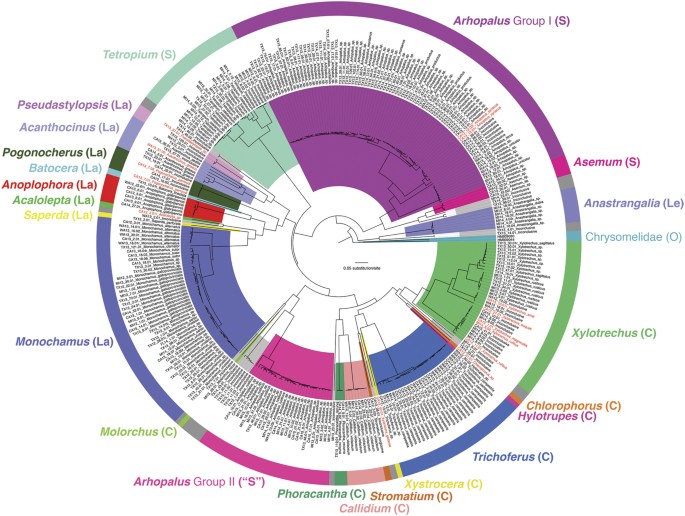The image is a detailed infographic centered around a large circle segmented into various colored sections, each labeled with specific names denoting different groups. Starting from approximately 12 o'clock and moving clockwise, the segments detail:

- Orthophallus Group 1 (S) in purple
- Asimum (S) in pink
- Anastrangalia in dark blue
- Chrysomelidae in light blue
- Xylotrexus in green
- Chlorophorus in orange
- Hylotrubase in purple
- Trichophorus in blue
- Xytrocera in yellow
- Stromatium in brown
- Colladium in pink
- Forocantha in green
- Orthophallus Group in darker pink
- Molarchus around 7 o'clock
- Monochemius between 8 and 9 o'clock
- Numerous smaller segments follow, including Seperida (yellow), Acoelolepta (green), Anoplophora (red), Batocera (blue), Pogonacheris (black), Acanthocinus (purple), Pseudodylopsis (light purple), and Tetraplum (green)

The interior of the circle mirrors the outer segments with corresponding colors and widths, divided further into smaller graphical sections. These segments are layered, with a multitude of detailed labels and numbers encircling the graphic. The core of the infographic is a white circle featuring minimal, uncolored graphs. The overall design is complex, with each segment and label meticulously detailed and color-coordinated to provide specific information about each represented group.